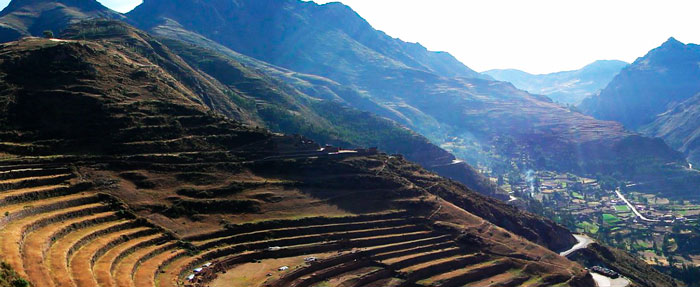This aerial photograph captures a panoramic view of a mountain range, featuring five prominent peaks with smooth, hazy summits. The foreground mountain exhibits distinctive terraced, stadium-like layers that resemble a theater with rows of seating carved into its brown, rocky slopes. The flat-topped peaks on the left side stand out prominently. The entire scene is bathed in bright sunlight, making the background appear white and obscuring fine details due to the glare.

In the valley below, a small village nestles among lush green trees and fields, interwoven with a network of roads. The roads wind sharply around the mountains and through the valley, yet no vehicles are visible. The verdant landscape lower in the valley contrasts with the rugged, rocky heights of the mountains. Despite the brightness of the scene, the intricate interplay of natural and man-made features is clearly visible, offering a glimpse into the serene yet majestic mountain environment.